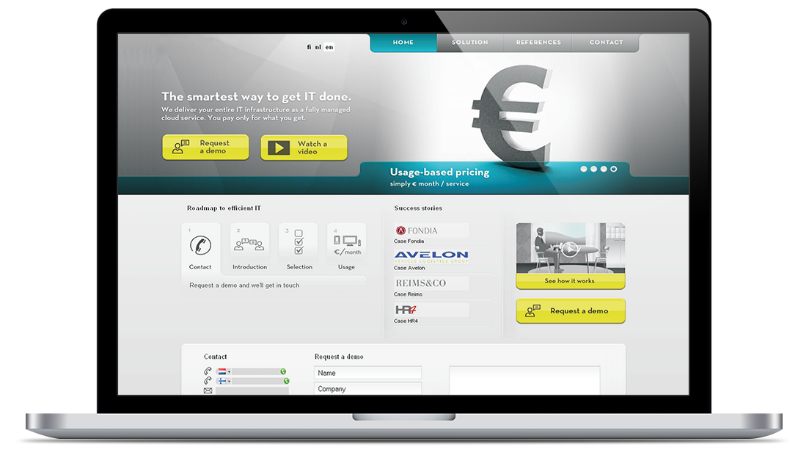The image depicts a laptop displaying a promotional webpage. The laptop has a silver bottom, and the screen content is framed within a black border. The upper portion of the screen features a gray background with bold, white text that reads "The smartest way to get it done." Below this headline is smaller white text, though its contents are not detailed here.

Beneath the text, there are two prominent yellow boxes. The first yellow box, located on the left, displays an icon of a person along with dark text stating "Request a demo." The adjacent yellow box to the right contains a video play icon and the words "Watch a video."

To the right of these boxes, a large circle with two vertical lines inside is shown, presumably a pause icon. Below this section, a blue banner intersects the screen with the text "Usage-based pricing. Simplify per month/service."

Following the blue banner is a light gray section. On the right side of this area, a title reads "Read map to efficient IT" with icons arrayed beneath it. One icon resembles a phone and is labeled "Contact." Another icon with two people is captioned "Introduction." There are also three buttons: two of them feature check marks, labeled "Selection" and "Usage," next to icons of a computer and a cellphone, respectively.

At the bottom of the gray section, there is a prompt saying "Request a demo and we'll get in touch." To the right of this text are some images and business names, which are not described in detail. The bottommost part of the screen provides contact information and repeats the "Request a demo" prompt.